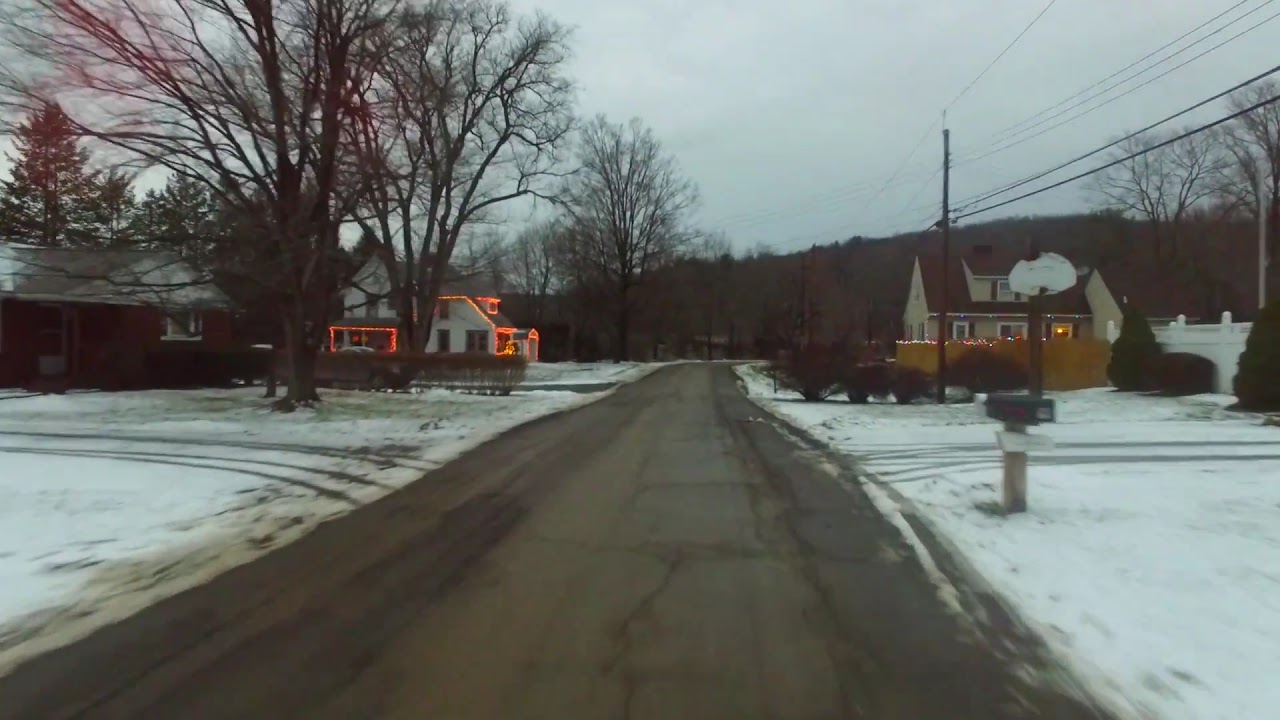In this image, we're looking down a slightly rough, dark asphalt roadway that recedes towards the center, where it disappears into a light hazy blue-white sky. Snow covers the ground on both sides of the street, though the road itself remains clear, revealing tire tracks where vehicles have pulled into driveways. At the bottom right corner, there's a black mailbox with a red flag. 

The street is lined with houses typical of a suburban neighborhood. On the mid-right side, there's a tan two-story house with a brown roof, adorned with Christmas lights on its wooden front porch. This house is surrounded by a variety of bare trees and bushes, characteristic of a winter scene. Directly in front of this tan house, but slightly towards the bottom right, there is a black asphalt driveway.

On the left side of the image, there's a white two-story house with a gray, pointed roof, and bright, colorful Christmas lights outlining the roof and awning. Behind this house, in the top left of the picture, there are evergreen trees standing tall against the snowy background.

Further back on the left, there's a one-story brick house partially obscured, adding to the quaint and cozy feel of the neighborhood. Straight ahead, beyond the houses, there's a view of a distant hill or mountain covered in trees, enhancing the wintery suburban atmosphere.